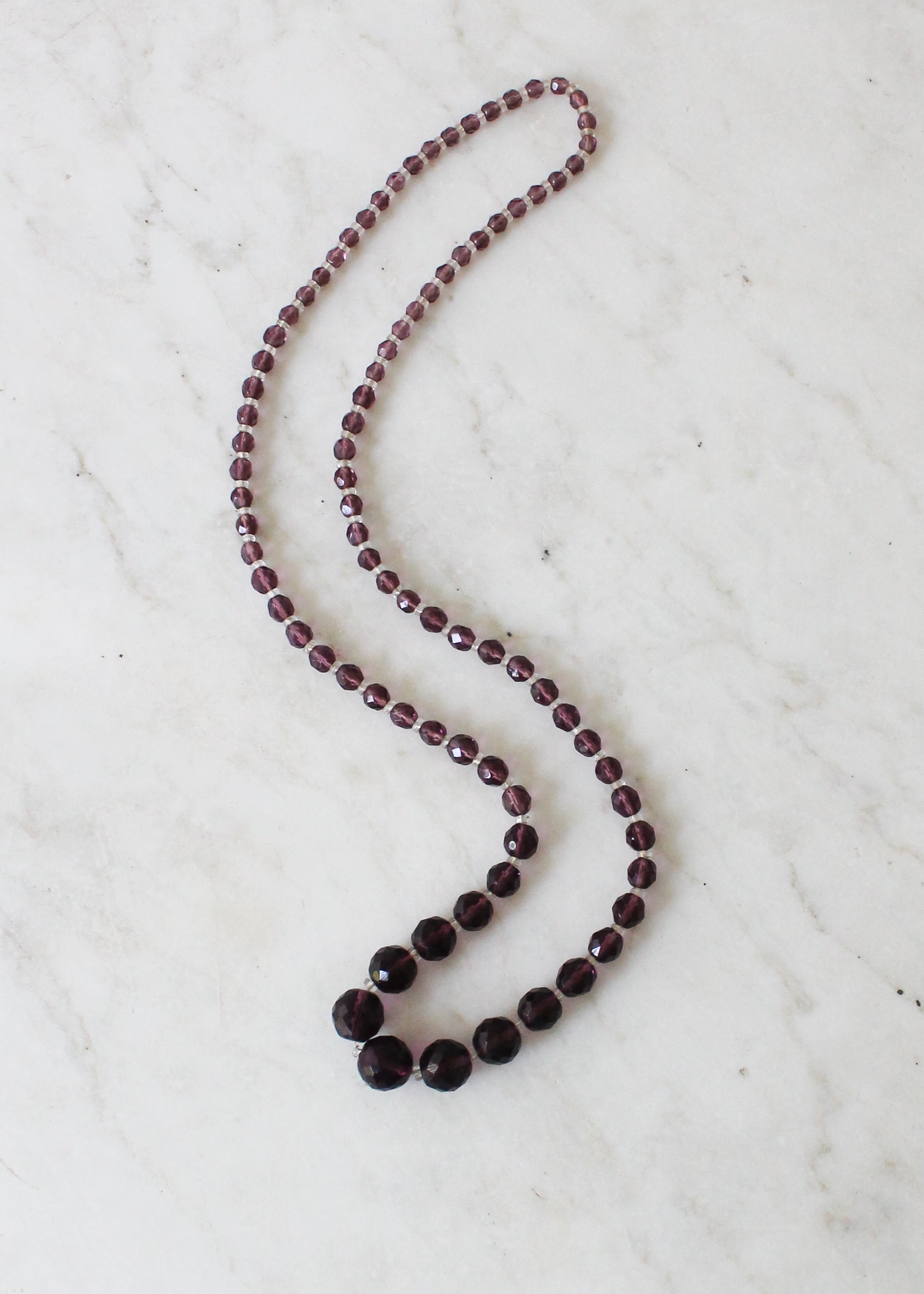The color photo showcases a striking necklace set against a grey-toned white marble background. The necklace, likely a piece of costume jewelry, features beads which may be quartz or plastic, strung together on a silver chain. The beads are arranged to form an S-shape, emphasizing the necklace's aesthetic appeal. Starting from the top, the smaller beads exhibit a light reddish-pinkish-purple hue, gradually darkening and increasing in size as they progress down the necklace. At the middle, where the necklace would typically rest on one's chest, the beads become notably larger and transition to a deep purple-red color, almost black. This detailed arrangement highlights the necklace's elegant gradient effect and subtle sophistication.